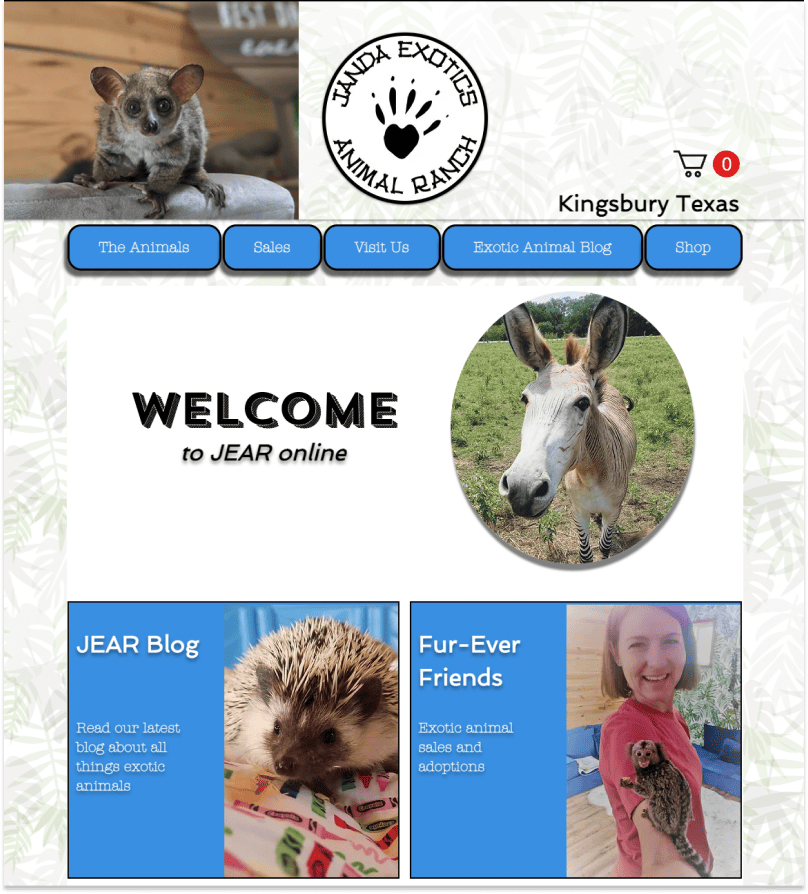This is a detailed screenshot from an animal website named "Janda Exotics." At the center of the image is the website's circular logo, with the text "Janda Exotics" written in a curved manner around the circle's top edge. Below the logo, it reads "Animal Ranch," and a paw print is situated between the words "Animal" and "Ranch."

To the left of the logo, there is an image of a lemur looking directly at the camera. On the right side of the logo, there is a shopping cart icon with a "0" indicating it is empty. Below this, the text "Kingsbury, Texas" is displayed.

Further down, five blue buttons provide different navigation options: "Animals," "Sales," "Visit Us," "Exotic Animal Blog," and "Shop." Just beneath these buttons, a welcome image states, "Welcome to JEAR Online," accompanied by a circular photo of a donkey.

Additionally, there are two more images below. One features an unidentified animal alongside text promoting their latest blog about exotic animals, titled the "JEAR Blog." The second image, labeled "Fur-ever Friends - Exotic Animals, Sales and Adoptions," shows a woman with an animal perched on her arm.